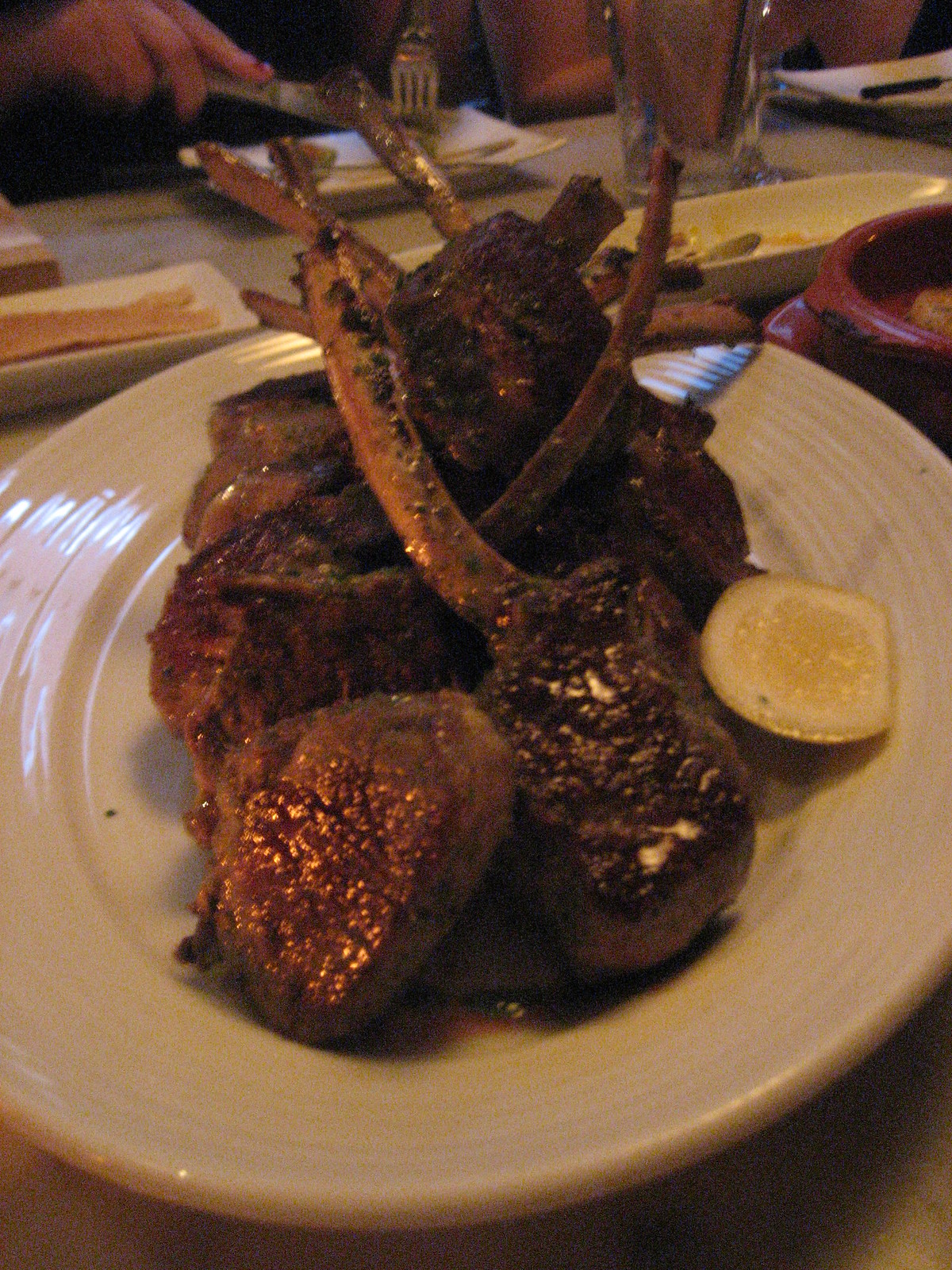This color photo captures a slightly blurry scene at a restaurant, creating a dim and atmospheric setting. The focus is on a thick ceramic white plate featuring what looks like a rack of lamb, possibly cut into lollipop-style chops where the meat is cleaned off the bone. The meat appears to be cooked rare, with visible traces of blood in the center. The lamb is adorned with a brown demi-glaze and crusted with green herbs near the bone area. A small slice of lemon accompanies the meat on the plate. In the background, there's a glass of water and additional plates, one of which may contain asparagus. A person with red nail polish can be seen cutting something with a knife and fork, though only their hands are visible. Overall, the image conveys a cozy, upscale dining experience, perfect for sharing on social media.